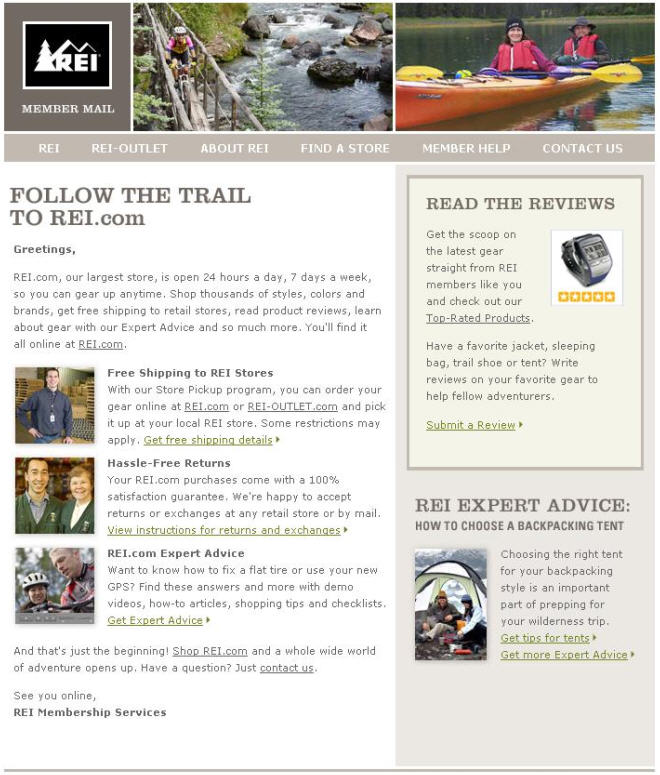This image is a screenshot taken from the REI website. At the top of the page is the REI logo, featuring a tree and a mountain emblem. Below the logo, the heading "Member Mail" is prominently displayed. The main content area of the image includes a scenic view of an individual riding a bike across a suspension bridge, framed by the natural landscape. Further down, a duo can be seen paddling together in a double-person kayak. 

The navigation menu lists several items in the following order: "REI," "REI Outlet," "About REI," "Find a Store," "Member Help," and "Contact Us." A banner toward the bottom of the image reads, "Follow the trail to REI.com," followed by a greeting and a paragraph of introductory text.

On the right-hand side, three icons depict additional features: "Free Shipping," "Hassle-Free Returns," and "REI.com Expert Advice." Further right, there is a prompt to "Read the Reviews." At the very bottom right corner, an advice section titled "REI Expert Advice: How to Choose a Backpacking Tent" is highlighted, likely offering useful tips for outdoor enthusiasts.